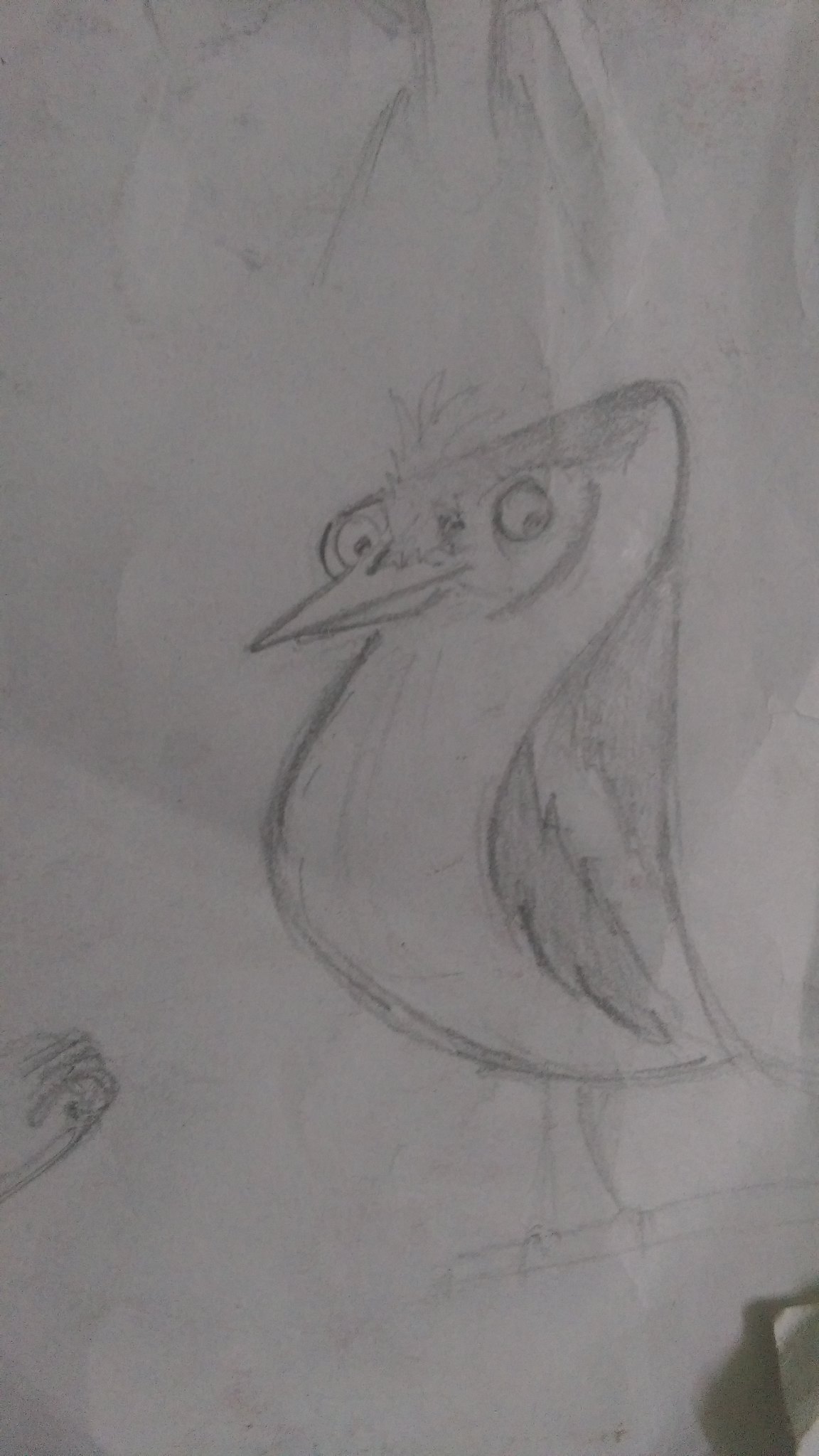This descriptive caption combines the detailed observations from all three perspectives:

In a photograph of a slightly creased piece of white drawing paper, there's an intricate black and white pencil drawing of a bird, likely a seabird, rendered in various shades of gray. The bird, positioned against a light indoor background, stands upright with a closed, sharply pointed beak and expressive, somewhat startled eyes that gaze directly at the viewer. A tuft of feathers grows between its eyes above its beak. The bird's head is flat on top, transitioning into an 'S' shape down its body to the wing, which curves delicately to mimic the breast's contour. On the bottom left side of the drawing, an ambiguous shape, possibly a foot or the end of a branch, is visible, while a similar indistinct form appears on the bottom right side. These elements, combined with the peculiar angles and creases in the paper, contribute to the overall striking and comical appearance of the bird.